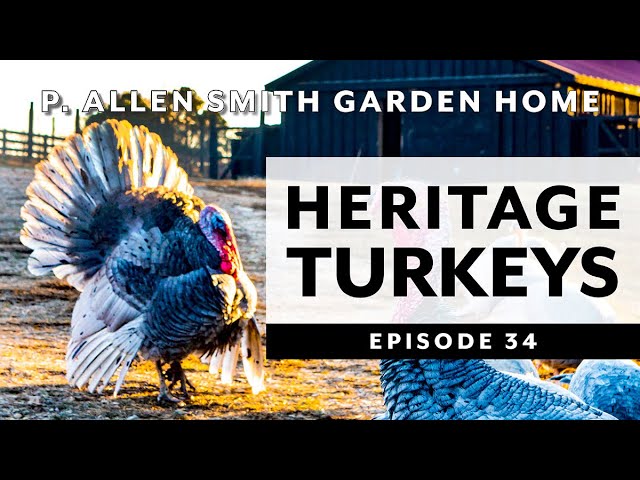The image appears to be the title slide for a video or a presentation related to "P. Allen Smith Garden Home." The title text, in white, is prominently displayed at the top of the image, with "Heritage Turkeys" in black text on a white field and "Episode 34" in white text on a black field overlaid in the middle. This color photograph features a large, impressive turkey on the left side, showcasing its abundant feathers and blue head with accents of white and gray. The turkey stands in bright sunlight on grassy ground, with a scenic farm setting in the background. There is a partially open barn or warehouse with a distinctive purple roof visible in the distance, framed by a fence and additional turkeys on the right side of the image. The overall impression is one of rural charm and focus on heritage turkey farming.